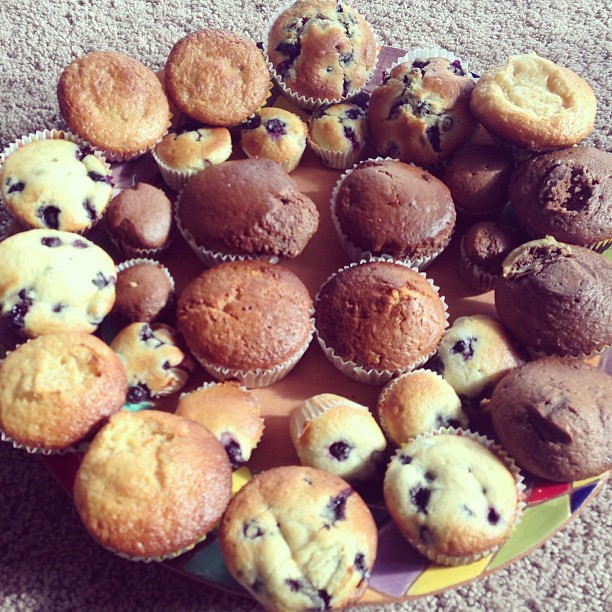This square snapshot photograph, taken from above, captures a variety of muffins arranged on a decorative porcelain plate. The porcelain plate has a stained glass-like rim featuring hues of purple, red, green, and yellow, and an orange-toned center. Large muffins, identified as blueberry, corn, and bran, form a circular pattern around smaller versions of the blueberry and bran muffins. In the very center, four muffins are grouped closely together. Each muffin is encased in a paper muffin cup. The plate rests on a light beige carpet, visible in the upper corners of the image. Despite being slightly blurred and of poor quality, the image is brightly lit, highlighting the various textures and colors of the muffins and the plate.